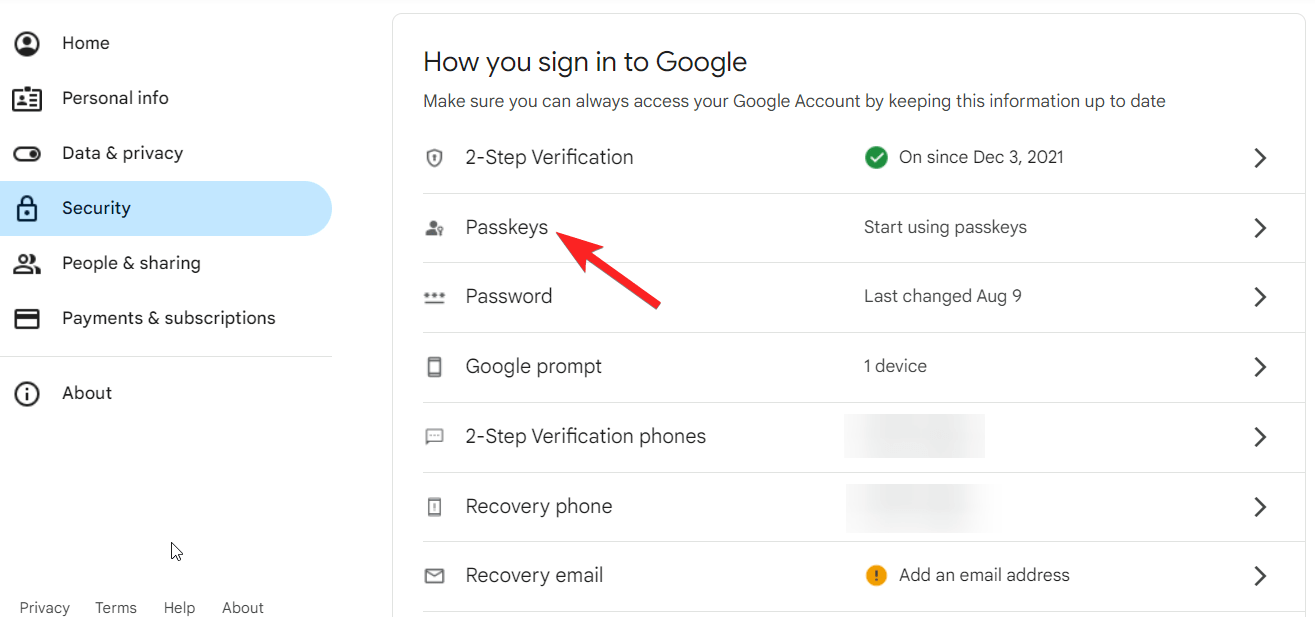**Image Description: Google Account Security Interface**

The image showcases a Google account security interface designed with a white background. On the left-hand side, there is a vertical navigation menu consisting of several sections:

- **Home Icon with a small person avatar**: This is located at the top.
- **Home with an image badge**: Directly beneath it, labeled "Personal Info."
- **Slider with 'Data & Privacy'**: Enclosed within a blue frame.
- **Lock Icon labeled 'Security'**
- **People Icon labeled 'People & Sharing'**
- **Credit Card Icon labeled 'Payments & Subscriptions'**
- **Circle with an 'i' labeled 'About'**
- The bottom left corner displays links in very small text: "Privacy," "Terms," "Help," and "About."

On the right-hand side, within a white rectangular box, black text reads: "How you sign into Google. Make sure you can always access your Google Account by keeping this information up-to-date."

A detailed breakdown follows:

- **Two-Step Verification**
- **Passkeys**: An arrow points to "Passkeys," coming from the bottom-right.
- **Password, Google Prompt, Two-Step Verification, Phone Recovery, Recovery Email**

In addition, on the right side:

- A checkmark indicating "On since December 3, 2021"
- Text: "Start using Passkeys"
- "Last login on August 9th, one device"
- **Two Grayed Out Sections**

An orange circle with a black exclamation mark contains the text: "Add email address."

Lastly, a white mouse cursor is visible at the bottom left, near the links in small text. 

This intricate layout offers users a comprehensive view of their Google account security settings.